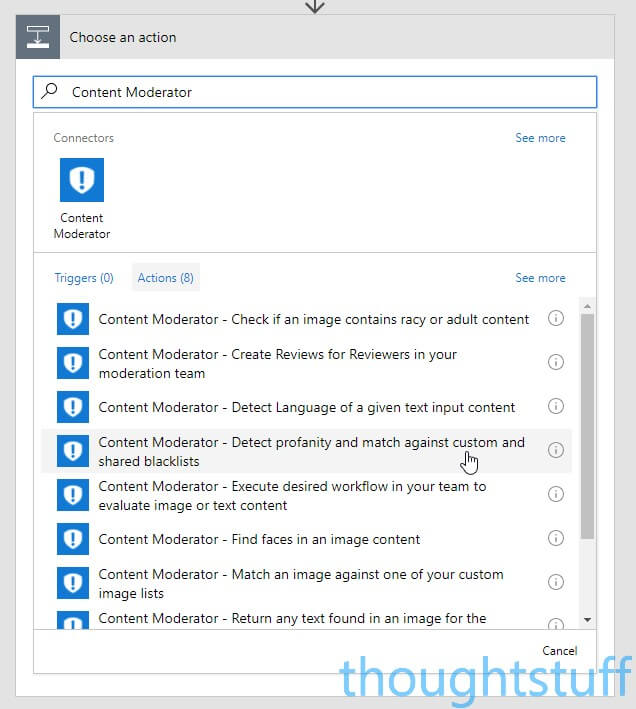A screenshot of a content moderation tool interface with a predominantly white and gray color scheme. At the top left corner, there is a drop-down menu presented with a square icon, allowing users to navigate through different sections. The background is mostly gray with a faint outline of a down arrow at the top.

The center of the screenshot features a search bar incorporating a magnifying glass icon. Next to the search bar, there is a blue shield icon labeled "Content Moderator."

In the middle of the interface, a detailed list of actionable items related to content moderation is displayed. These items include:
- Checking if an image contains racy or adult content.
- Creating reviews for the content creation team.
- Detecting the language of a given text input.
- Detecting profanity and matching text against a custom shared blacklist.
- Executing desired workflows within the team to evaluate both image and text content.
- Finding faces in image content.
- Matching images against custom image lists.
- Returning any text present in an image.

The right side of the interface has a scroll bar for additional navigation. Key phrases such as "Content Moderator" and the functionalities under it are highlighted in blue text. Edges of the interface are lined with thin gray borders, giving a structured appearance.

Overall, the interface is sleek and modern, designed to facilitate the tasks associated with content moderation efficiently.